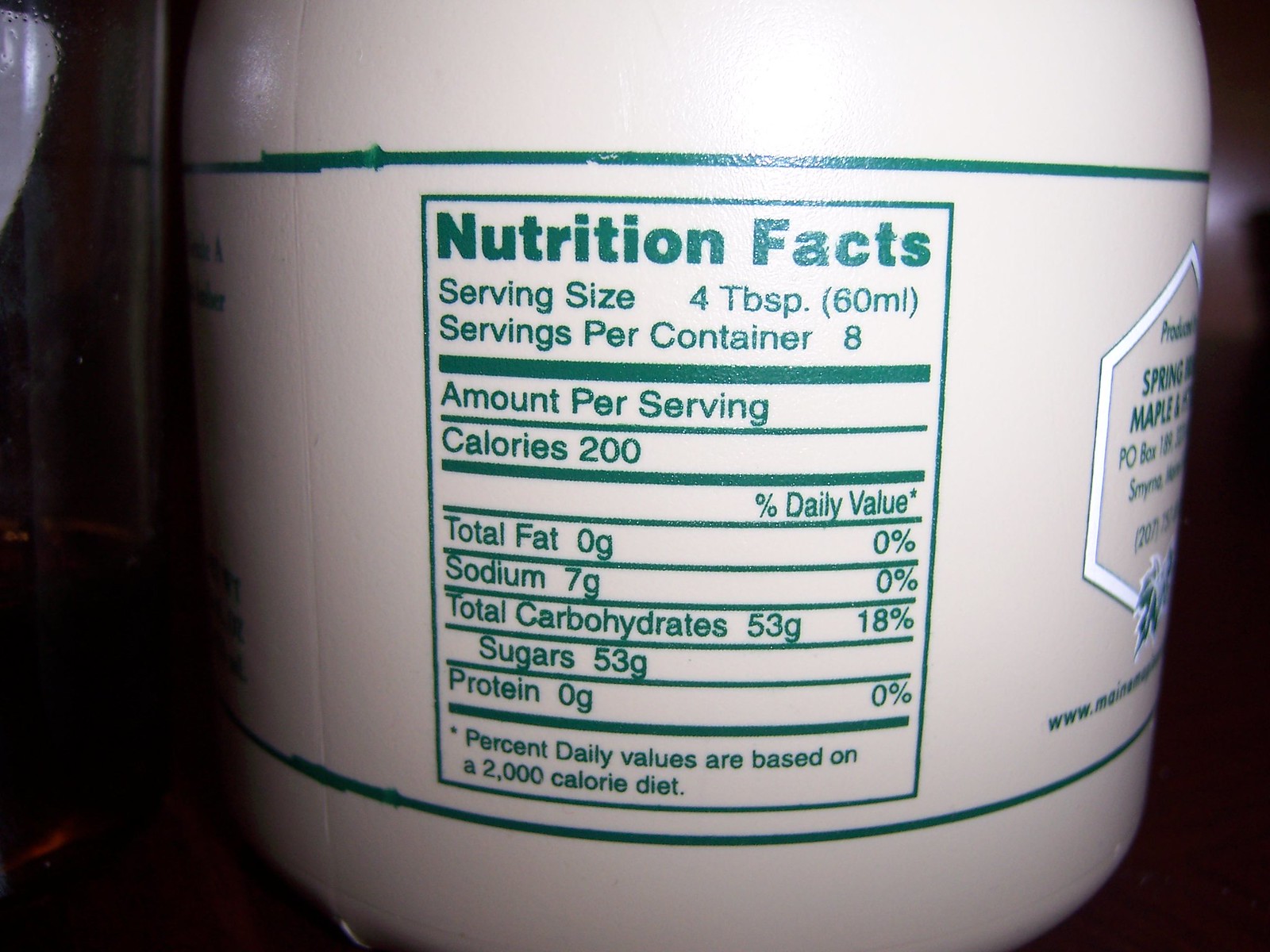The photo features a very close-up image of a white plastic jug of maple syrup against a dark brown to black background. The jug has green print accents: two small green stripes at the top and bottom. Dominating the image is the jug's nutrition label, which is partly visible. The nutrition facts display the following details: serving size of 4 tablespoons (60 milliliters), 8 servings per container, 200 calories per serving, 0 grams of total fat (0% daily value), 7 grams of sodium (0% daily value), 53 grams of total carbohydrates (18% daily value), 53 grams of sugars, and 0 grams of protein (0% daily value). Below, it notes that the percent daily values are based on a 2,000-calorie diet. To the right of the nutrition facts, there's a diamond-shaped white area with some text that is not legible. The labeling and nutritional numbers are all in green color. The jug appears to be placed on a very dark or black countertop with dim lighting, making the background appear almost black. The design and details closely suggest it is spring something maple syrup.